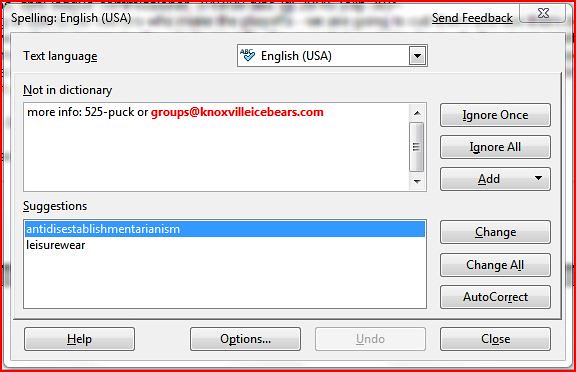This image captures a screenshot of a spelling check dialog box from a Windows computer. The dialog box, themed in colors of red, gray, black, and white, spans the entire image. At the top, it indicates the spelling language set to English (USA) and includes options for sending feedback and closing the dialog box via an 'X' button. The dialog box is analyzing an email address that is not in the dictionary—specifically "525-puck or groups at KnoxvilleIceBears.com."

Underneath the not found term, suggestions such as "anti-disestablishmentarianism," "terrorism," and "leisurewear" are provided as possible corrections. The interface offers multiple interactive buttons: "Ignore Once," "Ignore All," "Add" to dictionary, "Change," "Change All," "Auto-Correct," "Help," "Options," and "Close." Additionally, there is a grayed-out "Undo" button and an ellipsis representing more options. The detailed layout and the variety of available options indicate that this pop-up is designed for thorough proofreading and user convenience.